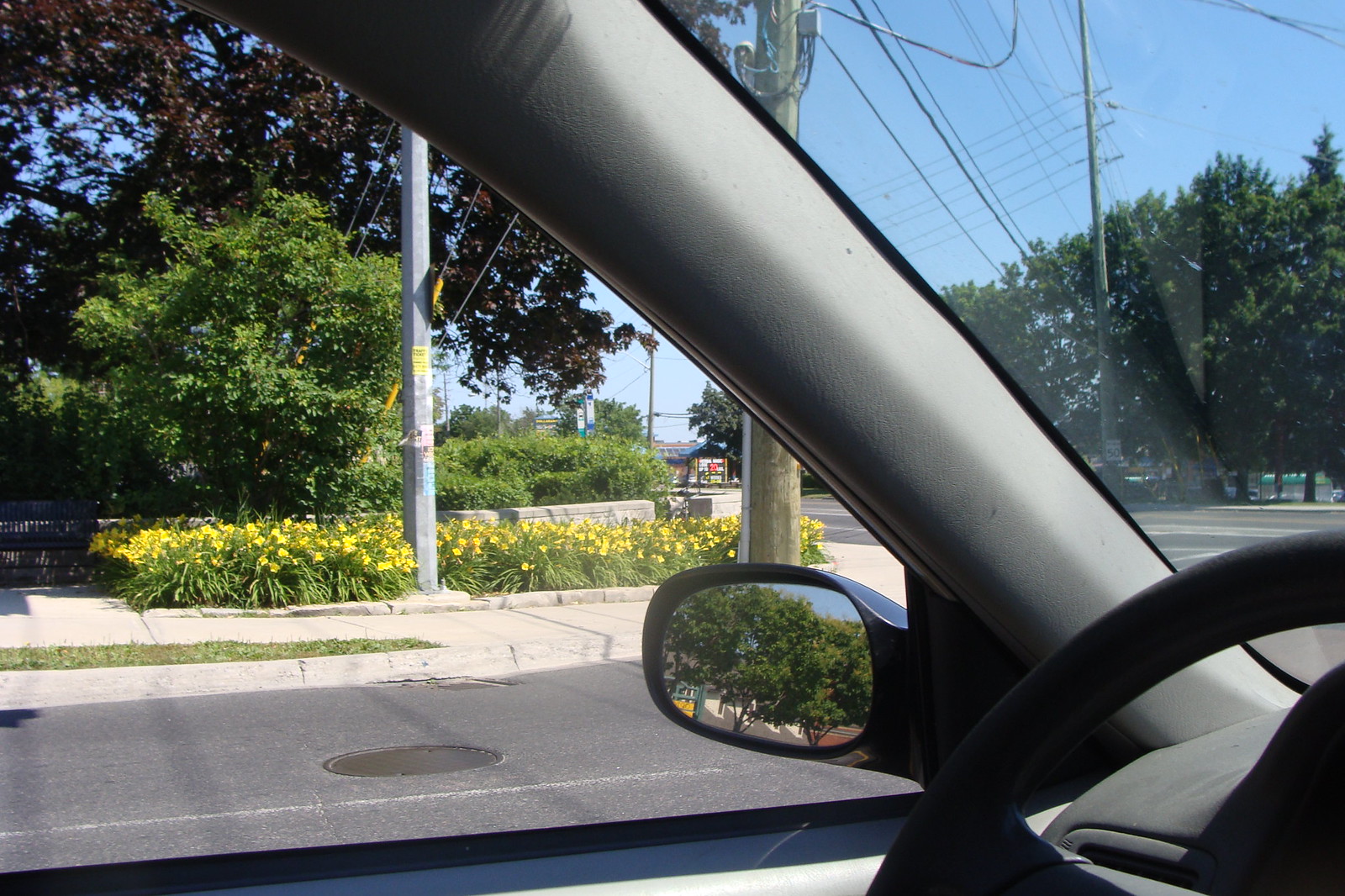The photograph is taken from the driver's seat of a car, offering a view through the driver's side window. The gray steering wheel and part of the dashboard are visible, along with the gray A-pillar framing the windshield and driver's side window. The rearview mirror, in black, captures the reflection of trees adorned with lush green foliage. Outside the car, a gray paved road stretches beneath a brown-colored round sewer grate. An off-white sidewalk runs parallel to the road, featuring a silver metal post and a brown wooden utility pole. The roadside is decorated with clusters of yellow flowers and lined with trees bearing light green leaves. In the background, trees with striking purple leaves add a pop of color to the scene.